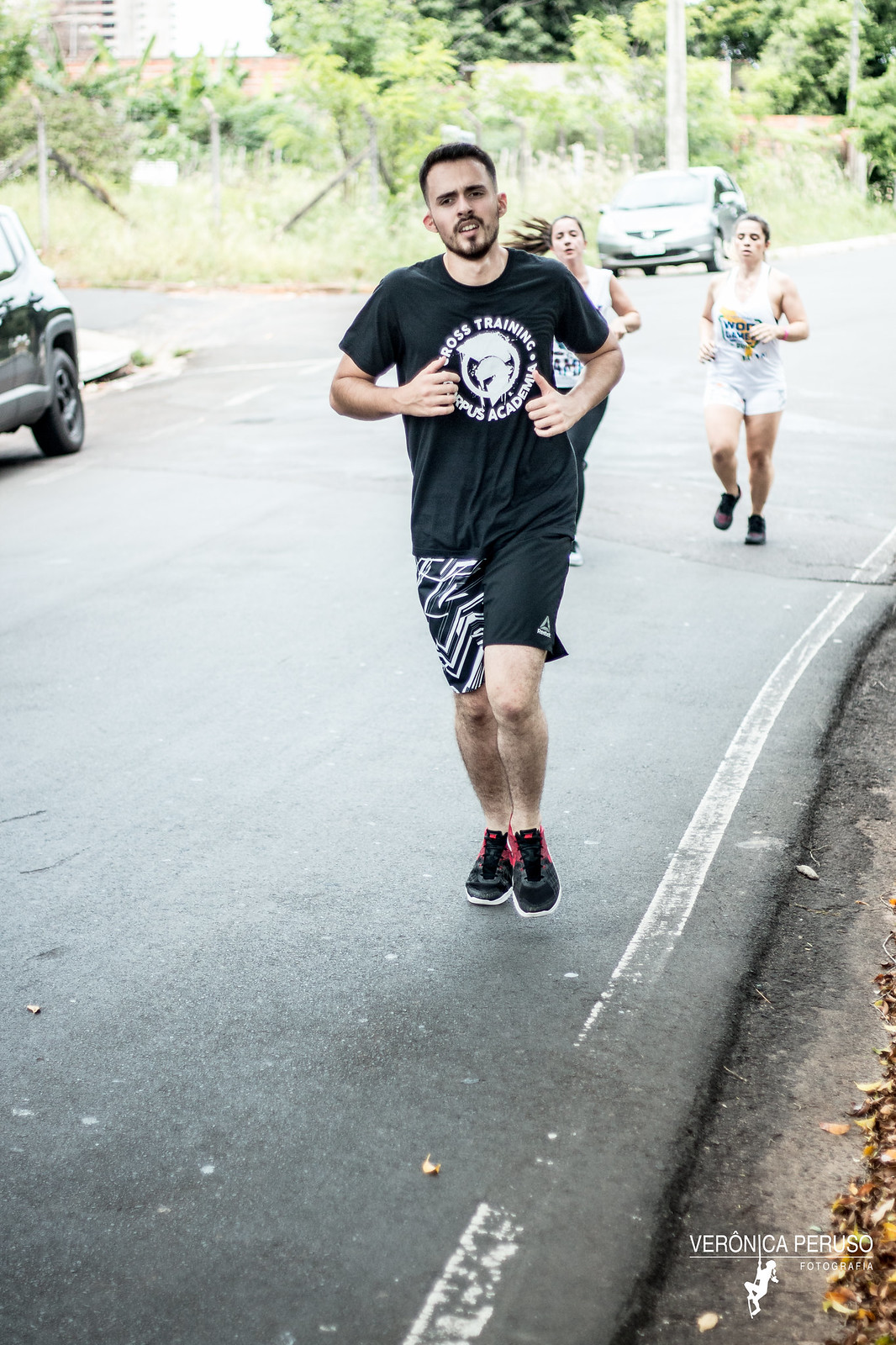This vertically oriented color photograph captures an energetic scene of runners, likely participating in a marathon or a street race. The focal point is a man in his mid-20s, sporting a black t-shirt with a distinctive logo featuring 'Ross Training' and a Spartan helmet within a circle, paired with black and white patterned shorts. His footwear includes black sneakers with prominent red stripes. Trailing slightly behind him are two women, both clad in white tops; the woman to the left wears black leggings, while the woman to the right sports white shorts and a tank top adorned with a 'World Game' logo featuring a yellow line and green accents.

The runners are making their way down a dark gray road marked by a faded white line along the edge, meeting a patch of dirt. In the backdrop, a gray van and another reflective, dark-colored car can be observed, along with a side road veering off to the left. This landscape is lined with light green trees and a mix of red and gray rooftops, interspersed with smaller, light green plants.

The photograph, taken on a bright, sunny day with a slight cyan hue, bears the watermark 'Veronica Peruso Fotografia' in the bottom right-hand corner. The watermark features an artistic logo of a woman climbing a rope, adding a unique touch to this vibrant, outdoor scene.